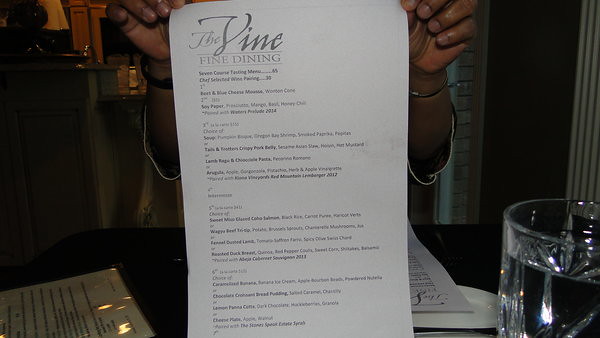The image features a detailed view of a menu from "The Vine," prominently displayed at the top in elegant gray cursive, labeled "Vine Dining" underneath. The menu, which is in gray text on a white background, has a narrow, elongated format. The text is too small to discern individual items. It is being held upright by a person's hands, with the fingers visible and the bottom of the palms showing. In the bottom right corner of the image, there is a glass pitcher, likely containing water. In the bottom left corner, a piece of paper with writing is slightly visible. The dimly lit background reveals indistinct objects, and another piece of paper is noticeable on the table behind the menu.